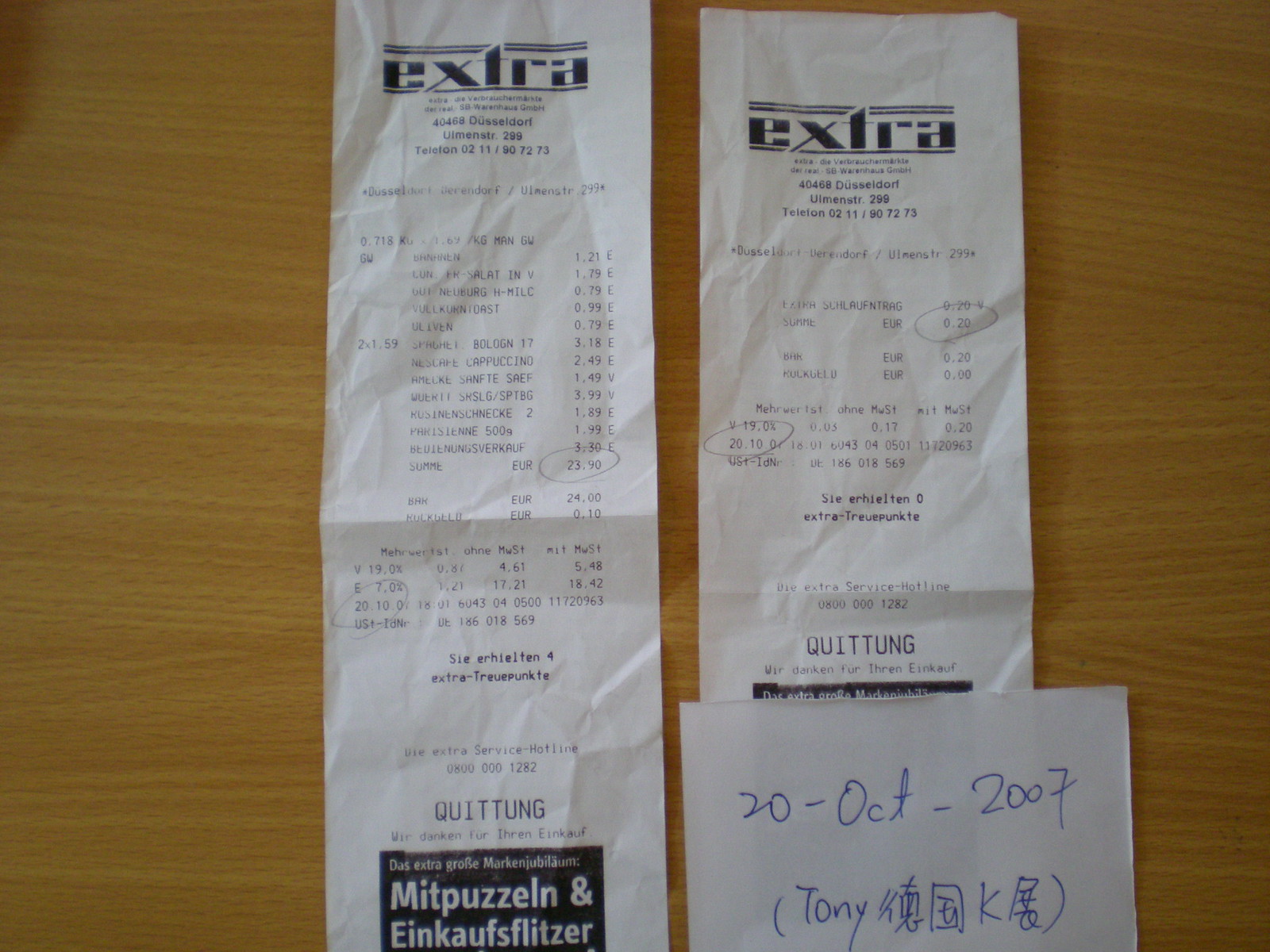This photograph captures two German receipts laid side by side on a faux wooden surface, characterized by visible grain and varying shades of brown. Both receipts prominently display "EXTRA" at the top in black letters with white borders, indicating they are from a store named Extra in Düsseldorf, Germany. The receipts suggest that the store is likely a grocery retailer, with itemized listings and prices. 

The receipt on the left features a fold across the middle, likely from being stored in a pocket. It shows a total amount of 23.90 Euros, with other circled numbers beneath it. The bottom of this receipt includes the words "Mitt Poulsen und Eikensflitzer" and "Wir danken für Ihren Einkauf," which translates to "Thank you for your purchase."

The receipt on the right also shows itemized entries, with circled amounts of 6.20 Euros and 20.10 Euros. At the bottom, it says "quittung," meaning "receipt," alongside a handwritten note on a small piece of paper that is superimposed on the receipt. This note, dated 20 October 2007, includes the name "Tony" followed by Chinese characters, all enclosed in brackets.

These details collectively emphasize the European, specifically German, origin and nature of the receipts, highlighting their connection to a grocery store in Düsseldorf.